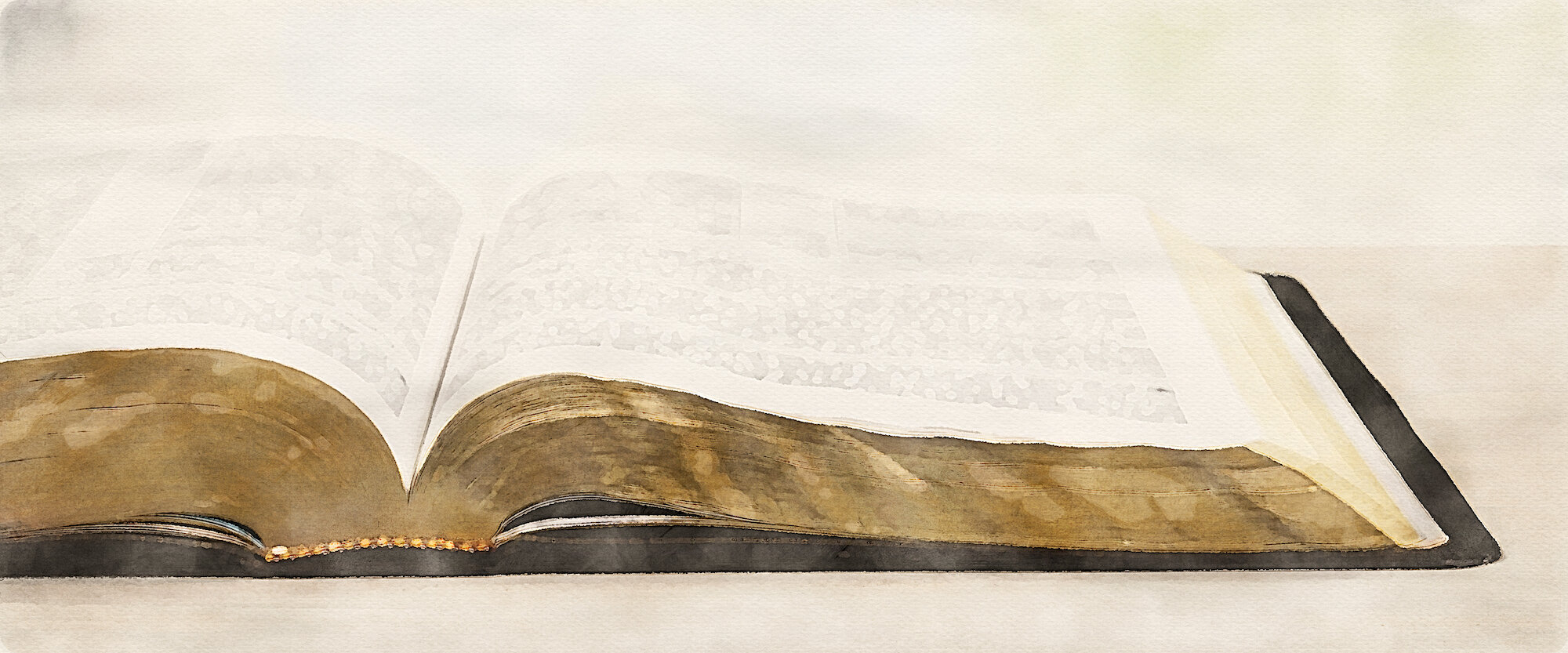This is a photograph of a large, ancient-looking book, potentially the Bible or New Testament, placed towards the left side of the image, yet centered vertically. The book, with a dark brown to black cover, is open to its halfway mark, revealing the full page on the right and a partial view of the left page. The white pages adorned with black text contrast with the golden edges, giving it an aged, distinguished appearance. It's resting flat on a white or very light-colored surface—possibly a table or tablecloth—with a bright, almost blindingly white background. The perspective is from the bottom edge of the book, emphasizing its width and the detailed texture of the binding, spotted with what look like water marks. The overall setting evokes a sense of solemn reading or reverence often associated with such volumes.